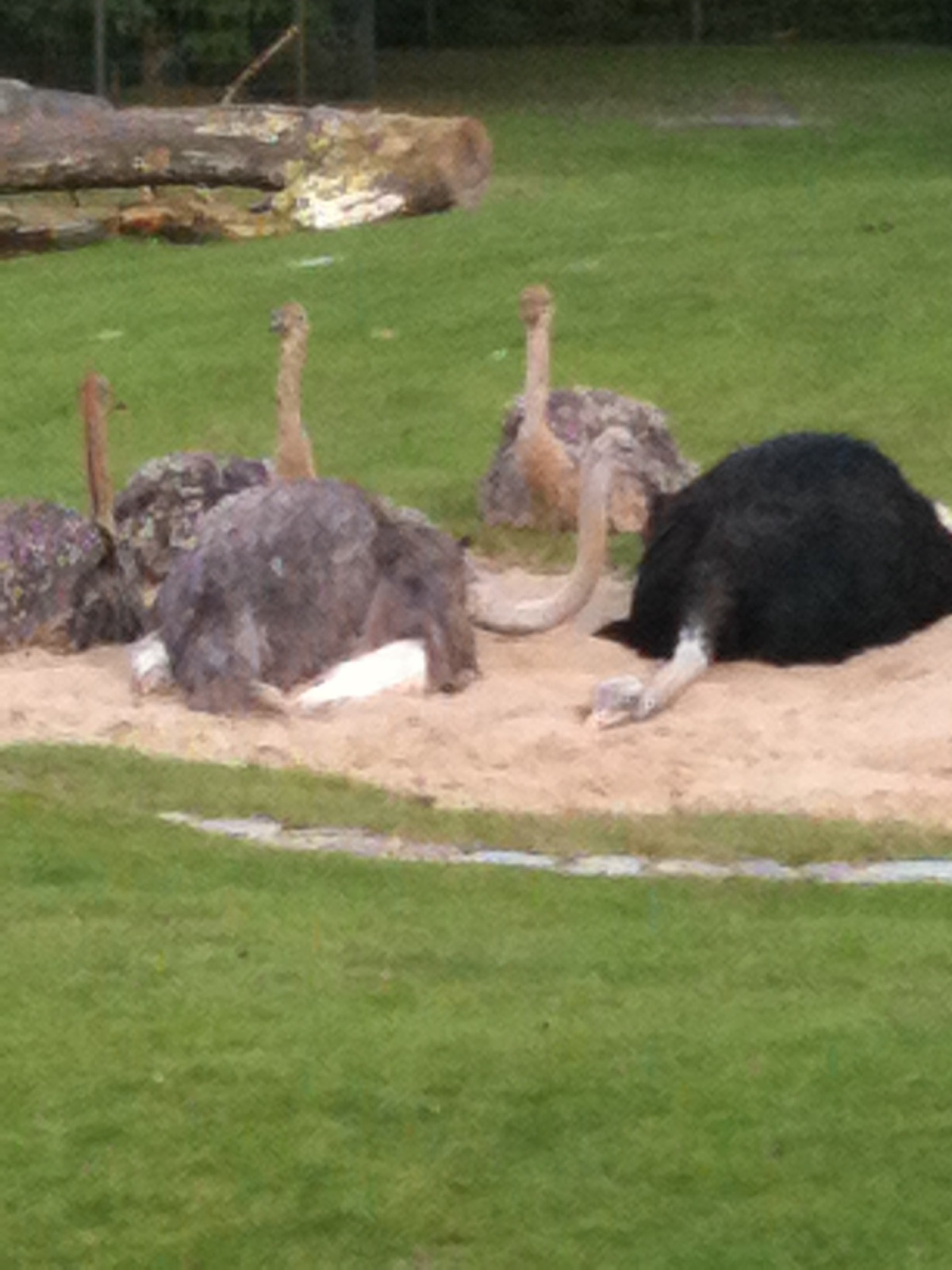The image depicts a group of five ostriches resting in a zoo enclosure on an overcast day. The enclosure features a well-kept grassy field with an oval-shaped sandy area in the middle. Four ostriches are lounging on the sand, while one is resting on the grass. The ostrich on the far right is a large black one with a white neck, light yellowish-orange beak, and closed eyes, appearing sound asleep with its head laying in the sand. Next to it, a dark gray ostrich with white fluffy legs and a bent neck looks down at the black ostrich. Behind them are three juvenile ostriches with downy, grayish feathers and tan necks, each with small black eyes and brownish-gray beaks. In the background, a large tree lies on its side, further emphasizing the enclosure's spaciousness. The overall scene is serene but slightly gloomy due to the cloudy weather.